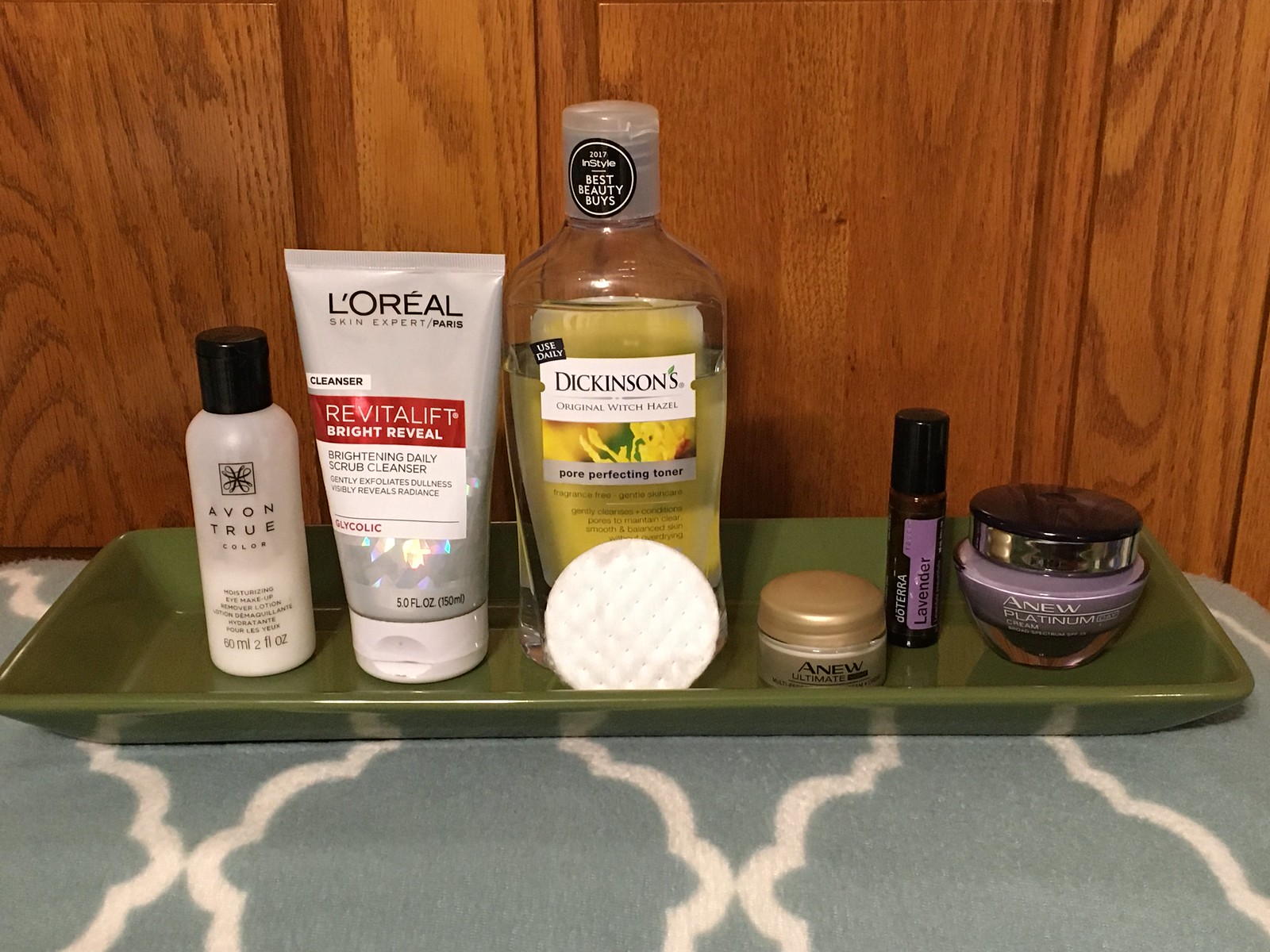The image depicts a gray carpeted floor, with a wooden wall featuring a grated design in the background. A green tray, reflecting the carpet, is placed on the floor and holds an assortment of skincare products. The carpet has a blue hue with white shapes adorning it.

On the tray:

1. **Left Bottle:** An Avon product, with most of its contents used. It features a unique square symbol with a flower made of four teardrops in a cross formation. The bottle holds 50 milliliters (or 2 fluid ounces) of a white liquid.

2. **Middle Item:** A L'Oreal cleanser, labeled "Skin Expert/Paris." The product details include a red square with white text stating "Brightening Daily Scrub Cleanser" and other descriptions, with a capacity of 5 fluid ounces. The container has a shiny, reflective, silver finish.

3. **Right Bottle:** Dickinson's Original Witch Hazel, marketed for its pore-perfecting toner properties. A sticker at the top proclaims it as one of the "Best Beauty Buys." Beside this bottle is a cotton pad.

4. **Lower Right Jar:** An Avon Anew Ultimate cream, housed in a brown jar with a lighter brown cap.

5. **Tube Next to Jar:** A black tube labeled with purple text indicating its lavender scent.

6. **Far Right Jar:** An Avon Anew Platinum cream, identifiable by its purple content and silver cap.

Overall, the scene provides a meticulously organized display of beauty and skincare products against a stylish backdrop.